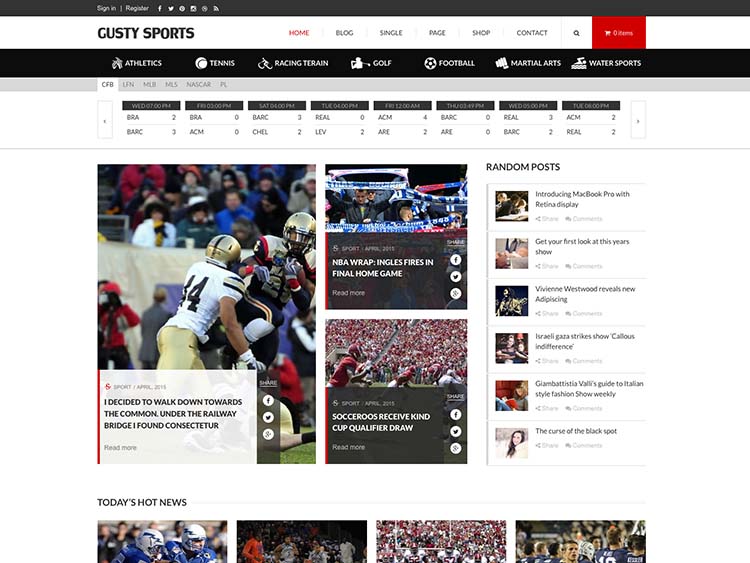The webpage displayed on the computer monitor is for "Gusty Sports." At the top, there is a black border featuring several options: "Sign In" and "Register" tabs, with icons for Facebook, Twitter, Pinterest, a clock, a Wi-Fi symbol, and two unidentified icons.

Below this, in a white section, the "Gusty Sports" logo is prominently displayed with navigational tabs including "Home," "Blog," "Single Page," "Shop," "Contact," and a search icon. Nearby, a red shopping cart icon indicates zero items.

A second black border showcases various sports categories: "Athletics," "Tennis," "Racing," "Terrain," "Golf," "Football," "Martial Arts," and "Water Sports."

Beneath this, a chart lists abbreviations for sports leagues or organizations: CFB, LN, MLB, MLS, NASCAR, and possibly PL.

In the main content area, images depict an NFL football game with a title adjacent, perhaps reading: "I decided to walk down towards the common, under the railway bridge, I found Consect Tour." A "Read More" link is provided.

To the right, two additional images feature:
1. An NBA game captioned "Rap, Ingles fires, and final home game."
2. Another NFL game with text mentioning "Soccer rules, receive, kind, qualifier draw."

Each article includes share buttons for Facebook, Twitter, and another unidentified platform.

Further down, a section labeled "Random Posts" highlights:
- "Introducing MacBook Pro with Retina Display."
- "Get Your First Look at This Year’s Show."
- "Westwood Reveals New Ad Pricing."
- "Israel, Gaza Strikes Show Callous Indifference."
- "The Curse of the Black Spot."

At the bottom, a section titled "Today's Hot News" appears, presumably featuring more sports-related content.